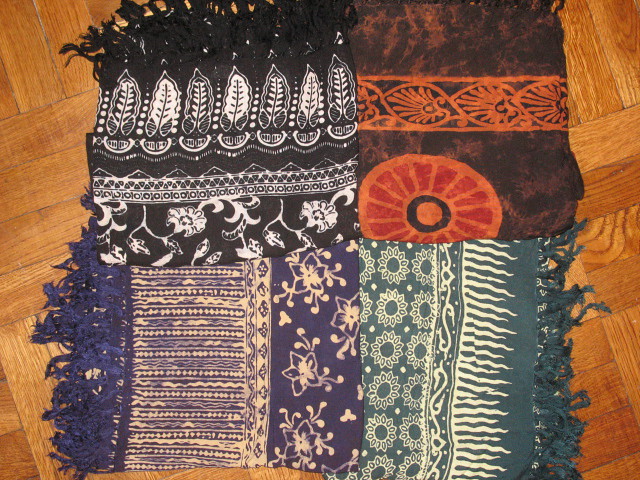This is a detailed photo of four folded textiles, possibly silk shawls or scarves, arranged in a two-by-two configuration on a reddish-brown parquet wood floor. Each textile features unique patterns and frayed edges, adding a frilly texture to their appearance. The top-left textile is black and white, adorned with leaves and flowers. To its right, the textile displays a neutral palette with orange, dark red, and brown hues, featuring a circular leaf pattern. At the bottom-left, a purple and blue textile showcases white flowers and intricate geometric designs. The bottom-right textile is primarily gray or off-blue with white flowers and geometric patterns. The consistent element among all four textiles is their frayed edges, giving them a distinctive, rustic look.